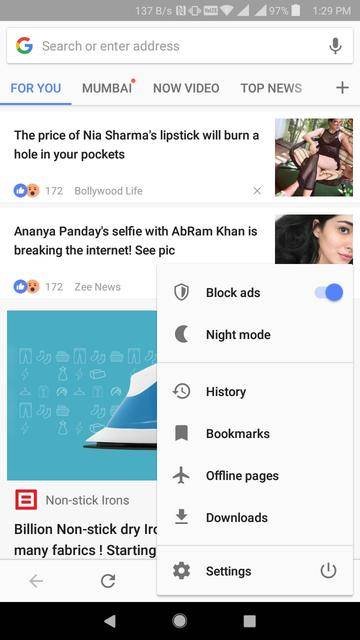At the top of the image, there is a long gray bar displaying a battery icon at 97%, nearly full and depicted in white. Adjacent to the battery icon, the time reads "1:29 PM." Below the gray bar, a search bar featuring the Google "G" logo and the text "Search or enter address" is visible. To the right of the search bar is a gray microphone or speaker icon.

Below this bar, there is a horizontal menu with the options "4U" in blue and underlined, "MUMBAI" in all capital letters with a small red circle beside it, followed by "Now," "Video," "Top News," and a plus sign.

Moving down, the first news headline reads, "The price of Nia Sharma's lipstick will burn a hole in your pocket," accompanied by a thumbnail image of a woman dressed in black, sitting outdoors on a chair. This is credited to Bollywood Life.

The next story features the headline, "Ananya Pandey's selfie with Abraham Khan is breaking the internet, see pic." Beside this headline is an image showing the left side of a woman's face with dark eyebrows and hair.

To the right of these stories is a long, vertical box starting with the label "Block ads," which is activated and indicated by a blue circle. Further down this menu are the options "Night Mode," "History," "Bookmarks," "Offline Pages," "Downloads," and finally, "Settings."